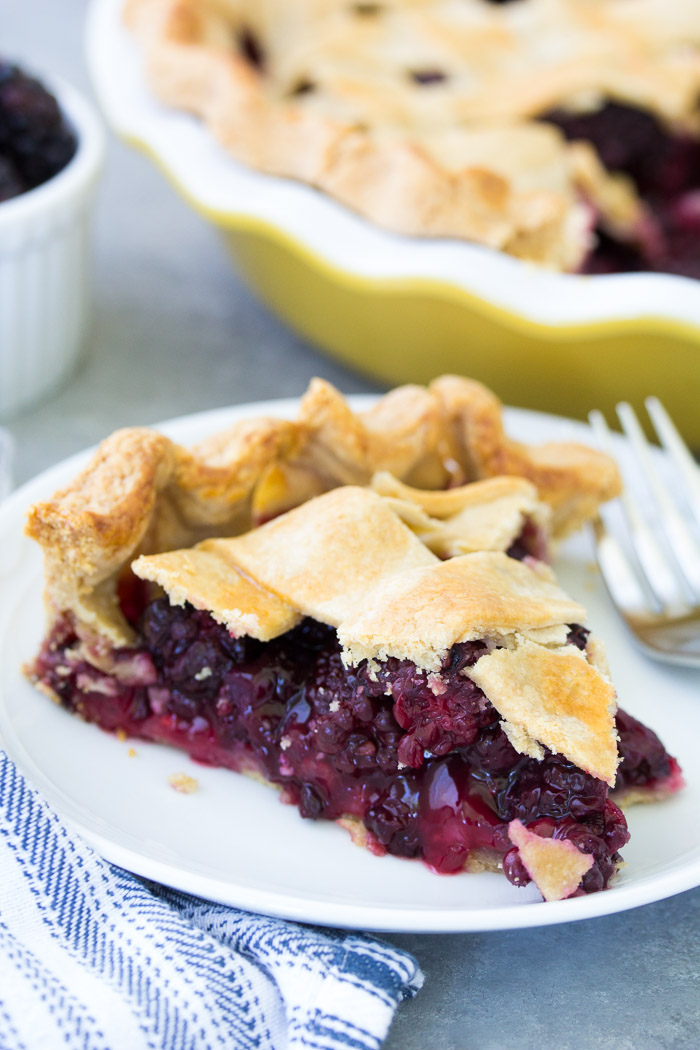In this photograph, captured in portrait orientation, a close-up of a piece of berry pie steals the focus. The slice, seated on a round white plate that stretches slightly off the image on both the left and right edges, is positioned lower than the center of the image. The pie, with its light brown ridged crust and dark purple filling—suggesting mashed berries or fruit—sits at an angle with the back in the upper left and the tip pointing downward to the right. A silver fork rests on the right side of the plate. A blue and white cloth napkin is partially visible on the surface to the left of the plate, extending off the frame. In the background, a blurred yellow pie dish, likely containing the remainder of the pie, is positioned behind the white plate, with a small white bowl to its left.